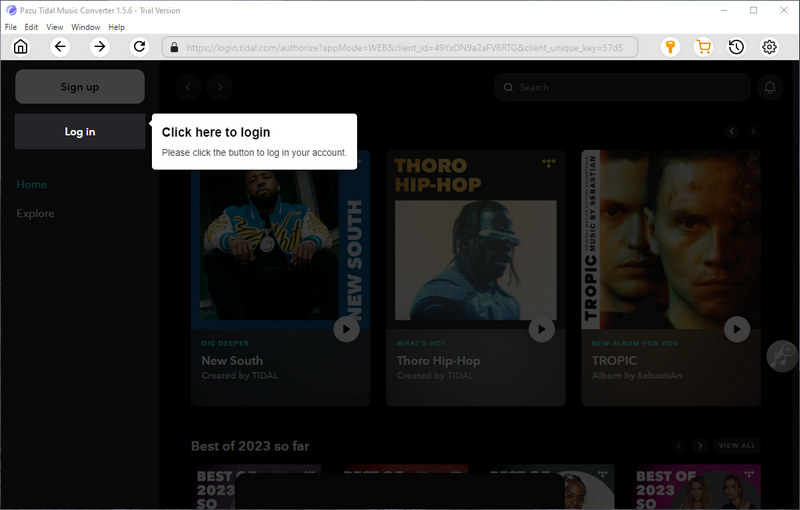The image displays a computer interface with a black background at the top, bordered in black. Below this, there is a white box featuring two concentric purple circles and some text. At the top of the interface, the menu options read "File," "Edit," "View," "Windows," and "Help," with minimize, maximize, and close buttons on the right side.

Underneath, there is a purple navigation bar containing several elements: a house icon, left and right arrow circles, a back arrow circle, and a search box. Additionally, the bar features a yellow key icon, a shopping cart circle, a clock circle, and a settings icon.

Beneath this navigation bar, the main content area has a black background. Prominently, there are two buttons—one for signing up and one for logging in. A large white box in this section includes the text "Click here to login. Please click the button to login to your account." 

Below this white box, thumbnail images are visible, which appear to represent different multimedia items. The images have titles such as "New South," "Thor Hip Hop," "Tropic," and "Best of 2023 so far," though some titles are partially cut off. Finally, at the bottom of the image, there is a large black box.